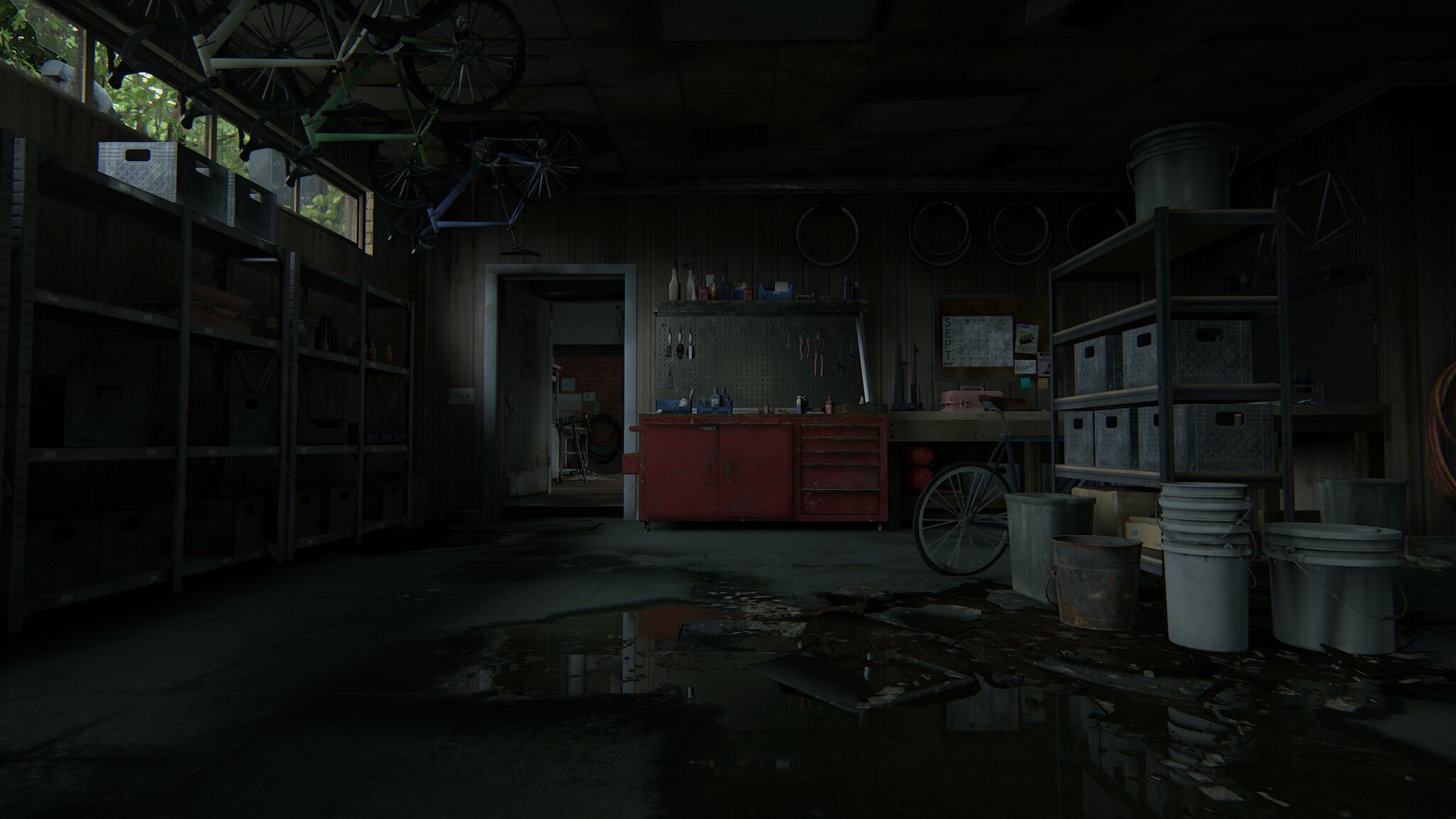The image depicts a dimly lit garage or workshop area. The floor is marked by a large, dark patch, suggesting a spill of water, oil, or tar. Several white commercial buckets, likely for cleaning or containing chemicals, are stacked nearby. A prominent red tool workstation with multiple drawers is visible, presumably housing various tools. Additionally, bicycles are hanging from the ceiling, contributing to the workshop atmosphere.